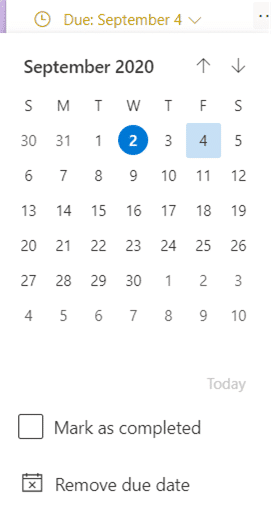The image features a calendar interface set against a stark white background. In the top left corner, there is a small vertical line in light purple with a light gray line beneath and to the right of it. Accompanying these lines is a brown clock icon next to text, also in brown, that reads "Due December 4th." On the far right side of the image, there are two dots, and above them is a downward-pointing arrow. 

Below this section, the caption "September 2020" is prominently displayed in bold black text, flanked by an upward-pointing arrow and a downward-pointing arrow to its right. The calendar layout below the text consists of seven columns labeled SMTWTFS, representing the days of the week. 

The dates for the month are arranged accordingly, with September starting on a Tuesday (the 1st) and concluding on a Wednesday (the 30th). The calendar also includes dates from the previous month (August) and the following month (October), covering the last three days of August and the first ten days of October.

At the bottom of the calendar interface, there are three clickable options: "Today," "Mark as Completed," and "Remove Due Date."